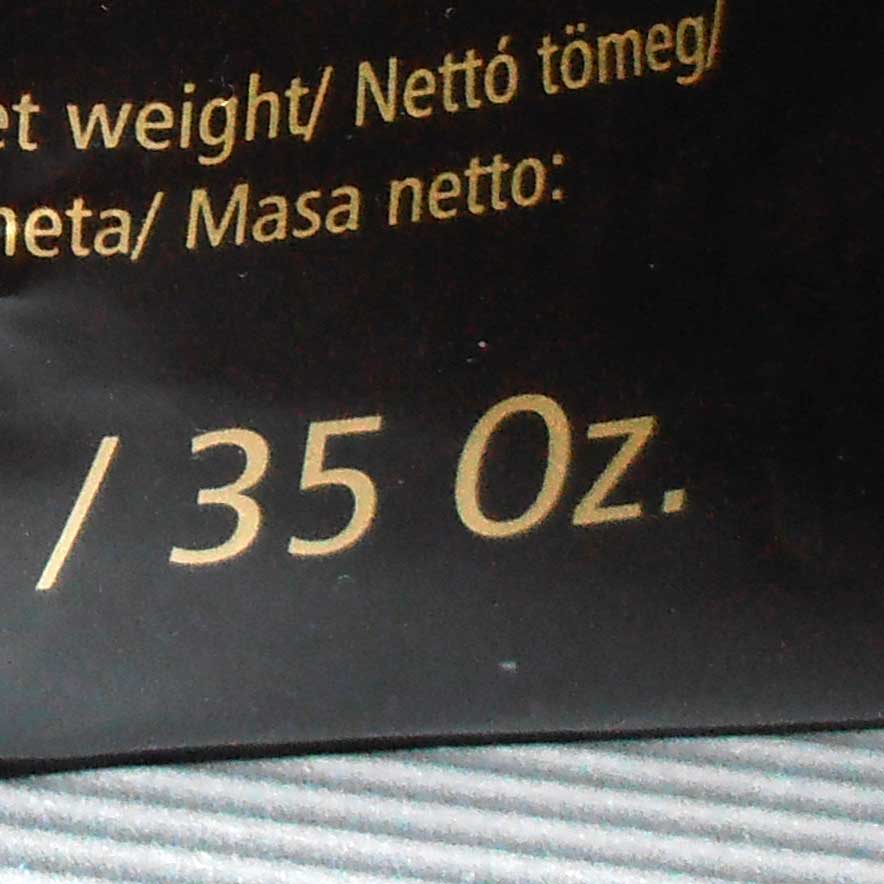This image depicts a highly zoomed-in segment of a black label with intricate gold text. The bottom portion of the label displays the measurement "35 OZ" in large gold letters, denoting 35 ounces. Above this, there are several lines of text, including the words "weight," "Netto," "Tomeg," "Meta," and "Masa," separated by slashes. The top part of the text is slightly cut off, but fragments of letters "E" and "T" are visible. This label appears to be sitting on a wavy, textured surface, possibly a white or gray material like carpet or a white towel, with some illumination enhancing the bottom part of the image. White specks are scattered across the label, giving it a slightly worn-out appearance.